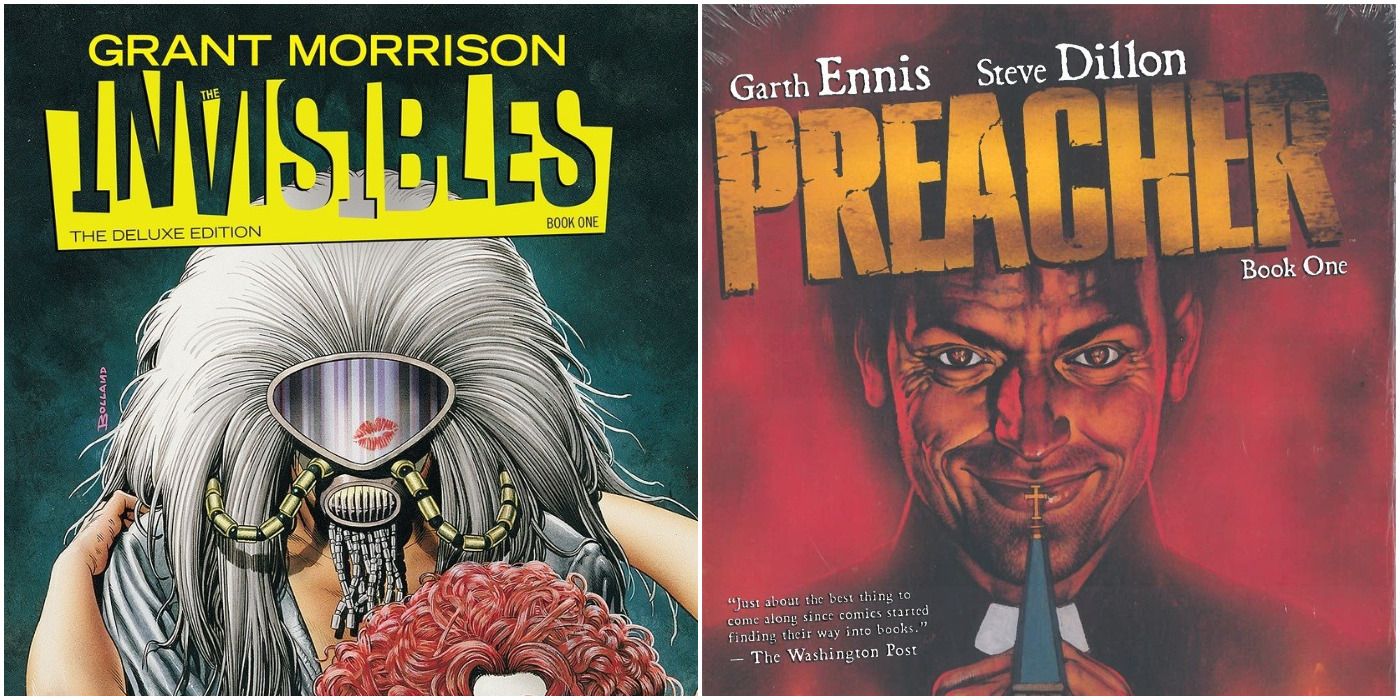The image showcases the front covers of two distinct comic books: "The Invisibles" and "Preacher."

On the left, the cover of "The Invisibles," titled "Grant Morrison, The Invisibles, the Deluxe Edition, Book One," features an enigmatic and surreal design. Against a predominantly black background, the title "Grant Morrison" is highlighted in bold yellow text, while "Invisible" is scattered in varying sizes. The artwork itself is peculiar: a central figure with curly red hair is positioned at the bottom right, reaching up behind them. Over their face is a silvery, reflective visor adorned with a red lipstick kiss mark. Attached to this visor are two tubes extending from its base, leading down to a grill-like structure with numerous dangling beads. The background of this cover is a strange greenish-blue hue, adding to the abstract and eerie aesthetic.

On the right, the "Preacher" comic book cover is drenched in dark red and black tones. The title "Preacher, Book One" stands out in bold yellow letters, with "Garth Ennis" and "Steve Dillon" noted above. Dominating the cover is an unsettling image of a man in preacher garb, sporting an ominous grin at the viewer. The background features a church steeple with a cross that aligns directly over the man's lips, reinforcing the dark and sinister theme of the comic. A quote from the Washington Post at the bottom left praises the work, calling it "just about the best thing to come along since comics started finding their way into books."

Both covers, while stylistically different, communicate a sense of intrigue and darkness, effectively inviting readers into the unique worlds created by their respective authors and illustrators.